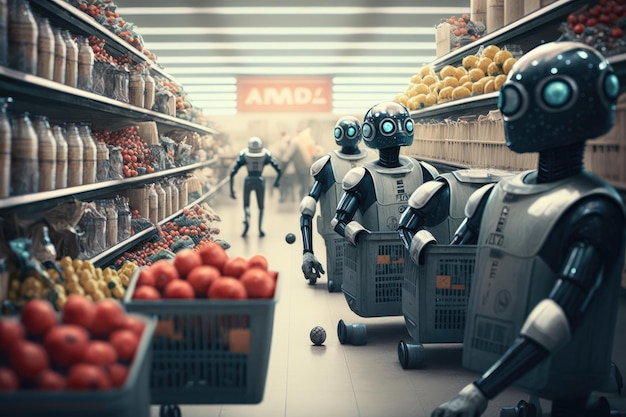In this hyper-realistic render, likely generated by a large language model, we are presented with a futuristic grocery store scene. The view captures an aisle flanked by shelves stocked with various items. On one side, the shelves primarily contain bottles, with a section displaying a pile of red fruit, possibly tomatoes. The opposite shelf features what could be manila file folders, and above them, tiers of yellow fruit, likely lemons and cherries, interspersed with more bottles.

Centrally, four humanoid robots are engaged in activities that resemble shopping or stocking shelves. These robots are distinguished by their floating platforms, akin to shopping carts without wheels. Three of the robots possess heads with at least three eyes that suggest a 360-degree field of vision, supported by narrow necks about four to six inches long. The fourth robot in the foreground, also headless, is an anomaly compared to the others.

In the background, another uniquely designed robot stands with no neck and its arms akimbo, seemingly surveying the scene. This robot adds to the complexity of the futuristic setting. Two balls lie on the floor, and one of the humanoid robots appears to be picking one up, adding a dynamic element to the scenario. The detailed depiction of the robots and the setting, with emphasis on the unconventional floating carts and multi-eyed robots, captures a vivid and intriguing glimpse into this imagined future.